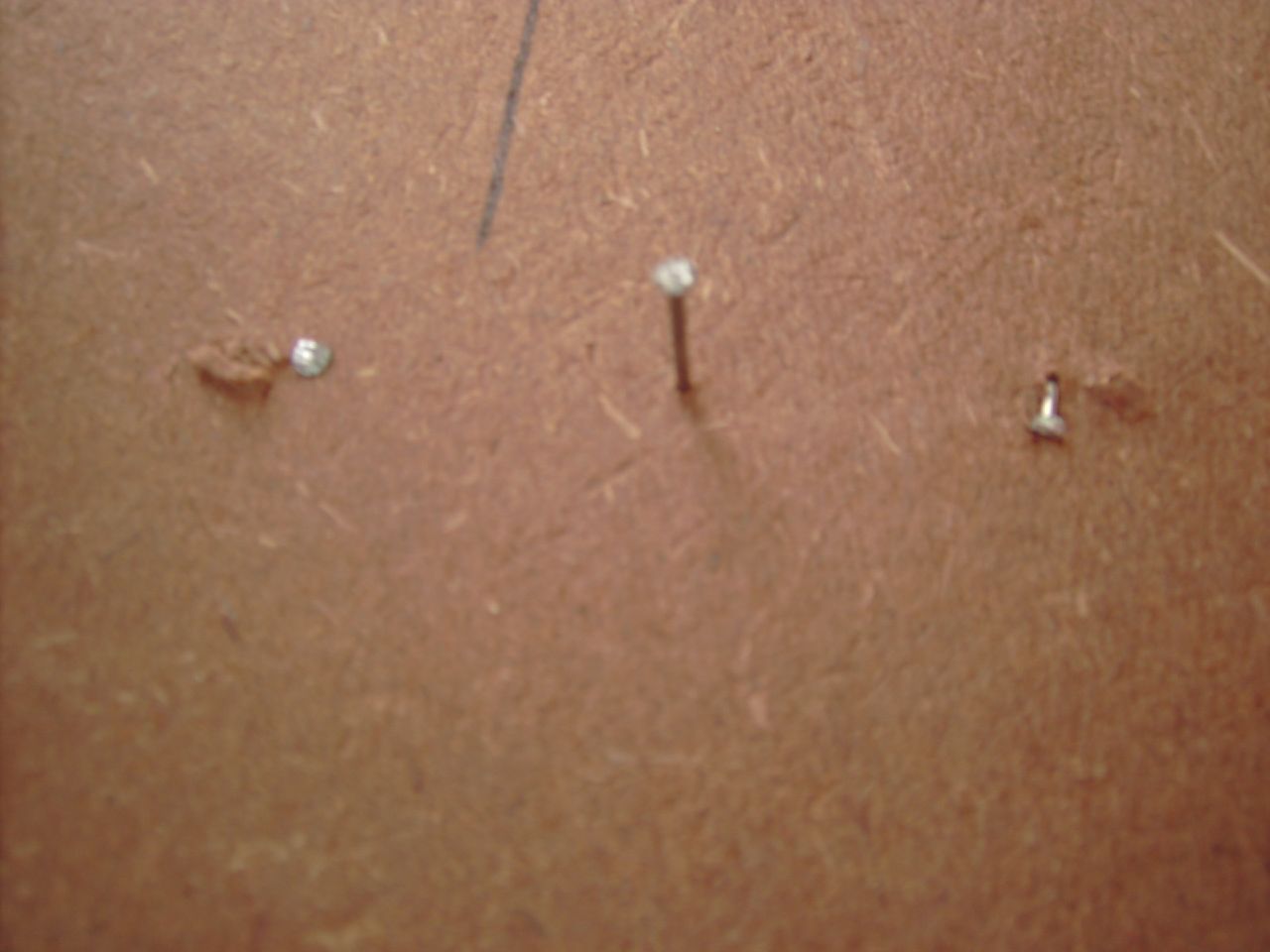The image showcases a highly magnified view of a light brown cork board-like surface with a cluster of three metal nails arranged in a row across the top middle section, each spaced about two inches apart. The first nail on the left is hammered in but bent sharply mid-way, with part of the head embedded at an angle. The second nail in the middle stands out about an inch from the surface, barely nailed in, revealing both its shaft and head prominently. The third nail on the right is driven all the way into the board. Adding to the detail, there's a black line, possibly made with a marker or ink pen, located between the second and third nails toward the top. The surface also features small, white streaks, suggesting wear or previous use, including a faint mark near the first nail, indicating where another nail might have been removed.